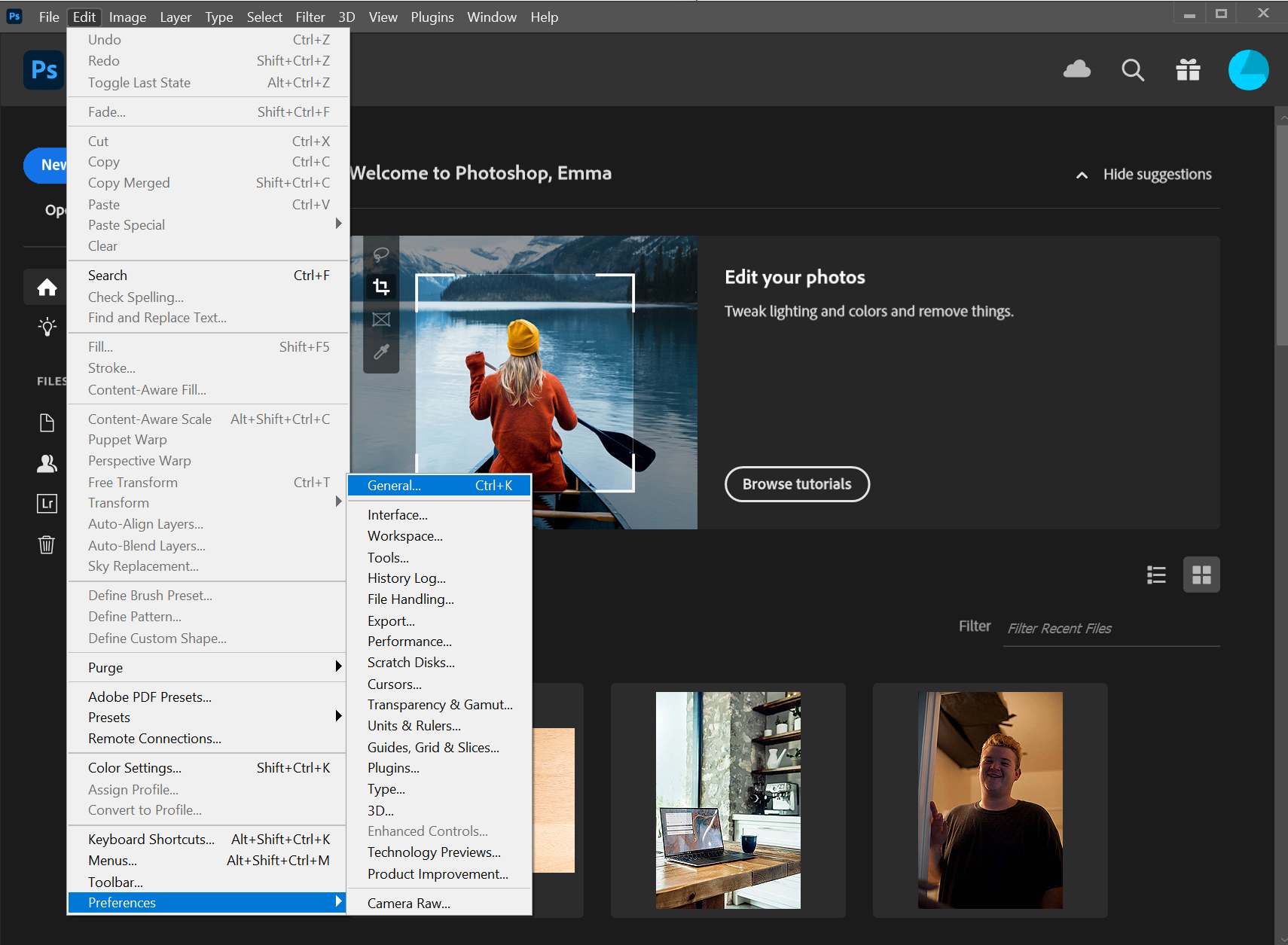The screen displays an image search page with a black background, featuring a welcoming message: "Welcome to Photoshop, Emma." Below this, it reads "Edit Your Photos," accompanied by a stock photo of a woman in a red sweater and yellow hat, rowing a sailboat on clear blue water towards distant mountains. The cropping icon is selected, highlighting the crop tool's functionality.

Beneath this, two additional images are visible. The first photo shows an open window, a laptop, and a drink on a table. The second image portrays a person, with a detailed dropdown menu on the left side offering various options such as: redo, toggle, fade, cut, copy, copy merge, paste, paste special, clear, search (highlighted in a darker color), check spelling, find and replace text, fill, stroke, content-aware, content-aware scale, puppet warp, perspective warp, free transform, auto-align, and more.

To the right of this dropdown, a smaller box presents a comprehensive list of categories, including: general interface, workspace tools, history log, file handling, export performance, scratch disk, cursor, transparency and gamut, units and rulers, guides, grid and slices, plugins, type, 3D enhanced controls, technology previews, product improvement, and camera raw.